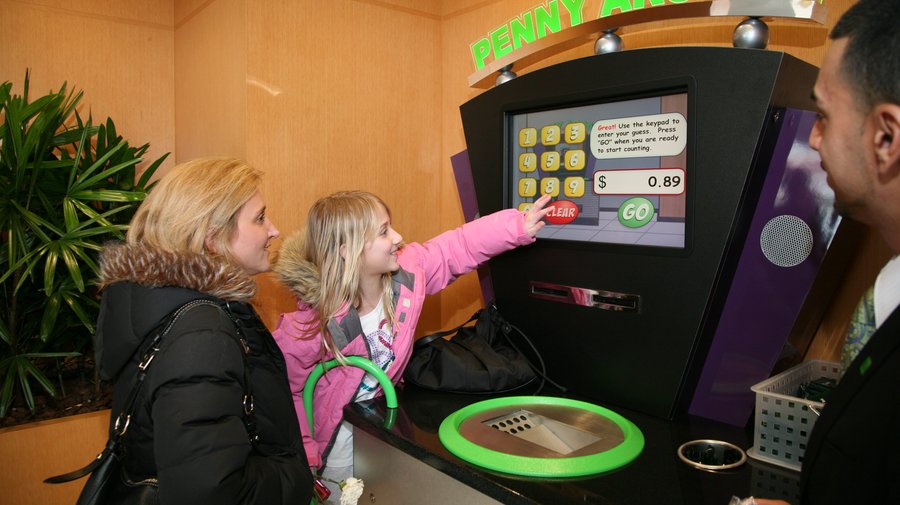This photograph, taken indoors against a background of light brown walls and faux green plant decorations, depicts a family engaged with a coin-counting machine labeled "Penny Arcade" in green letters. Central to the image is a black, triangular-shaped machine with a touch screen currently displaying instructions and an amount of 89 cents. The touch screen features a yellow keypad, a red clear button, and a green go button, accompanied by a green coin slot at the base. To the left, a blonde mother with light skin, dressed in a black coat with brown faux fur trim and a black purse over her shoulder, stands smiling. In front of her is her blonde daughter, approximately 10-12 years old, wearing a pink coat with similar fur trim. The daughter, also smiling, reaches out to touch the screen. On the far right side, partially visible, is a darker-skinned man with short black hair, donning a black suit and green tie, observing the interaction with a slight smile. The warm, indoor atmosphere and the detailed expressions suggest a light-hearted family moment centered around the coin machine.